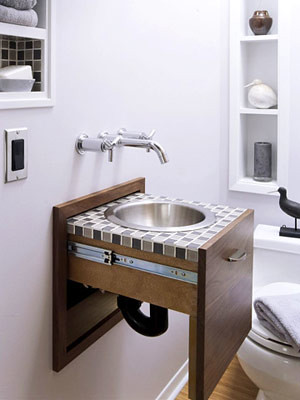This image showcases a uniquely designed, compact bathroom that exudes cleanliness and modern appeal. The standout feature is a distinctive sink, the true centerpiece of the room. The sink is ingeniously built into a cabinet drawer, providing a sleek and multifunctional aesthetic. The sink bowl is a silver basin set into a tiny countertop adorned with a checkerboard pattern. The drawer part is designed with a metal bar mechanism to enable smooth opening and closing, revealing a black pipe underneath that recedes into the wall when the drawer is shut.

The front of the sink drawer features a brown wooden panel with a silver handle, adding a sophisticated touch. Mounted on the wall above the sink are three unique control handles—two for hot water and one for cold, all white with silver ends—alongside a spout, all arranged in a linear fashion.

Adjacent to the sink, on the left, is a bar-style light switch, and above that, two small cabinets. The top cabinet houses neatly folded towels while the lower one stores a square object. Both cabinets feature a decorative pattern that complements the sink's checkerboard design.

In the background, there are three small shelves, each decorated with a distinct item: a long gray candle on the bottom shelf, a round, white object resembling a fat duck on the middle shelf, and a bronze cup-like item on the top shelf.

The image also captures part of a regular white porcelain toilet, partially in view with a towel casually placed on its seat. Atop the towel sits a black duck figurine, adding a playful touch to the bathroom's decor.